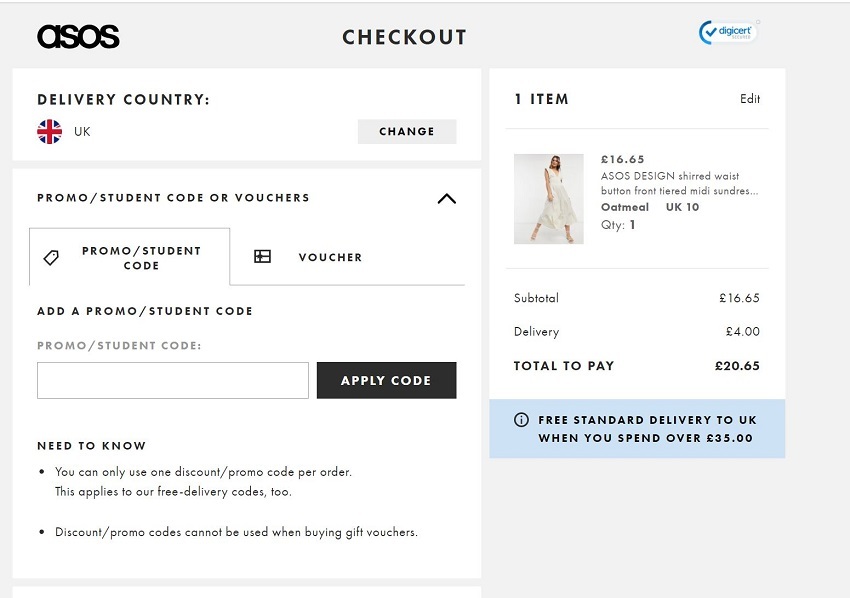Screenshot of the checkout page on the ASOS website. The delivery country is set to the UK, with an option to change it via a "Change" button. The overall design consists of a combination of light gray and white colors, with black font used throughout. A section for entering promo, student codes, or vouchers is available, where users can input a code and click the "Apply code" button to the right. Below this section is a note specifying that only one discount or promo code can be used per order, including free delivery codes, and that these cannot be applied when purchasing gift vouchers.

On the right side of the page, details of the item in the cart are displayed: an ASOS Design shirred waist button front tiered midi sundress. The sundress, shown worn by a model, is white and labeled "oatmeal" in color, available in size UK 10. The subtotal for the order is £16.65, with additional delivery charges not specified.